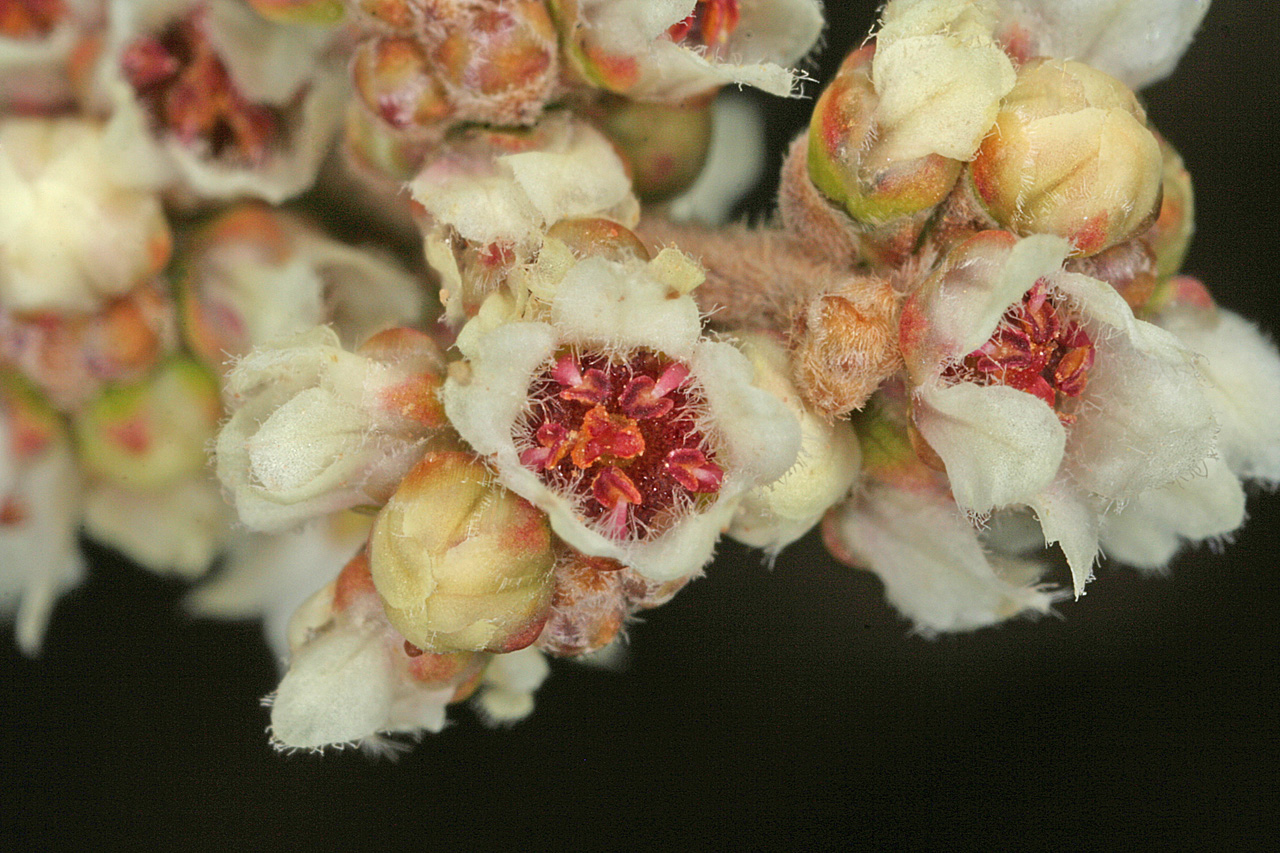This photograph on a black background showcases clusters of unknown vegetation, possibly flower buds or plant structures, in various stages of opening. The buds are tightly packed and exhibit a spectrum of colors, ranging from white and tan to green, red, and a touch of orange. The buds, resembling folded artichoke leaves or soft, feathery material, present a mix of tightly closed forms and partially open ones, with some displaying dark red stamens in the center. The overall appearance includes whitish hues, greenish tones, and some brownish areas with a fur-like texture on the edges. The lack of labeling adds to the mystery of the plant's identity, making it a captivating and intricate subject of natural development.